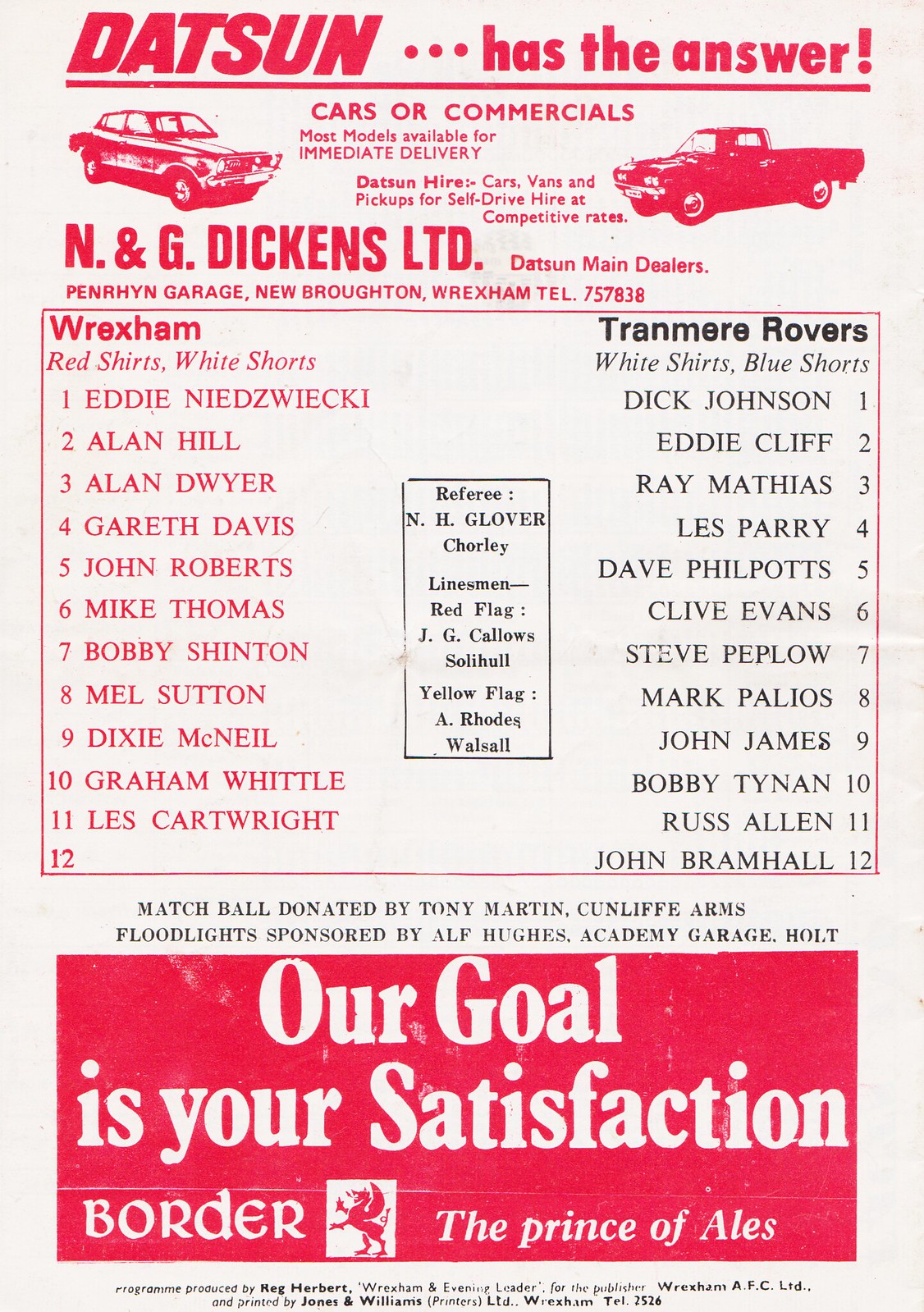This vintage poster features a white background with red lettering prominently stating, "Datsun has the answer." Flanked by images of a car on the left and a pickup truck on the right, the text below highlights Datsun's offerings: "Cars or commercials, most models available for immediate delivery" and "Datsun hires cars, vans, and pickups for self-drive hire at competitive rates." Further details include "NNG Dickens LTD, Datsun Main Dealers, Ferron Garage, New Broughton, Wrexham, 757838."

Centrally placed on the poster are team listings for a sports match. On the left side, in red, "Wrexham," noted for wearing red shirts and white shorts, with a list of 11 players. On the right side, in black, "Tranmere Rovers," described as wearing white shirts and blue shorts, with a list of 12 players.

Additional text at the bottom of the poster reads: "Our goal is your satisfaction," encased in a red box alongside "Match ball donated by Tony Martin, Cunliffe Arms, floodlights sponsored by Alp Hughes, Academy Garage Holt." The poster also features the phrase "The Prince of Ales" next to an image of a mythical winged horse, symbolizing a bygone era.